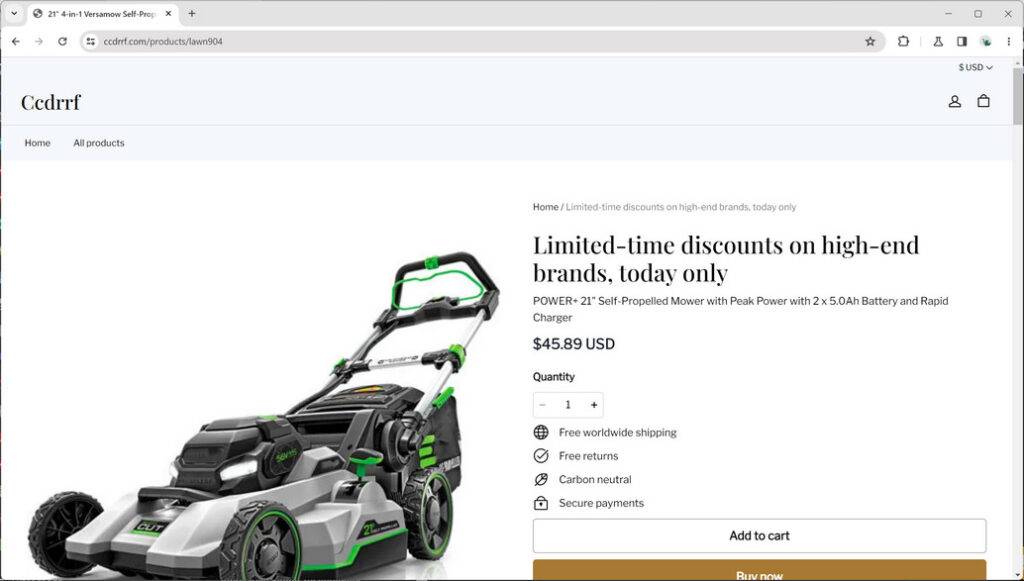The image features a product page for a high-end lawnmower branded as "CEDRRF," with the text "HOME" displayed beneath it. The page showcases various details about the lawnmower, which is silver and black with neon green-highlighted parts, and includes a bag attachment. Prominently featured is a banner reading "Limited Time Discounts on High-End Brands Today Only." The product itself is a "Power 21 Self-Propelled Mower with Peak Power," which comes with two 5.0AH batteries and a rapid charger, priced at $45.89 USD for one unit. It also advertises perks such as free worldwide shipping, free returns, carbon neutrality, and secure payments. The bottom section of the page includes two buttons: "Add to Cart" and "Buy Now," the latter in a goldish-brown color with white text. Above all this, the breadcrumb navigation reads "Home / Limited Time Discounts on High-End Brands Today Only."